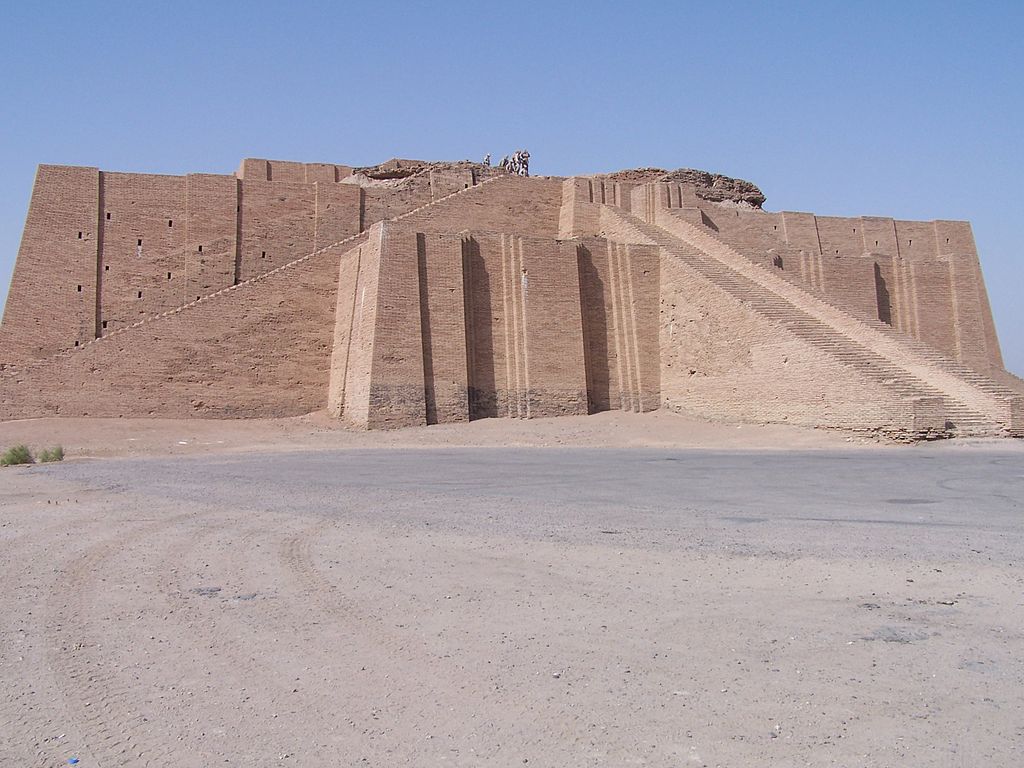The image is a color landscape photograph of the Great Ziggurat of Ur in Iraq, captured in clear daylight under a cloudless blue sky. The central subject is the large, multi-story rectangular structure made from brownish-beige brick or stone, showing signs of wear over time. Dominating the scene are two symmetrical staircases ascending on either side of the ziggurat, leading to the top where a small group of tourists, archeologists, or visitors are present. The building is positioned centrally, surrounded by a foreground of hard-packed sand and gravel interspersed with small arid plants. Additionally, a paved turnaround section of asphalt is visible coming in from the right side, contrasting with the dusty, beige surface. There is no text or border within the image, emphasizing its realistic and representational depiction of this ancient architectural site.